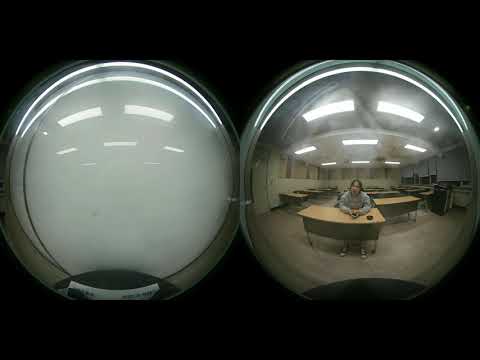The image features two equally sized circles placed side by side against a pitch-black background, resembling scenes viewed through a fisheye lens or a peephole. The circle on the left is bordered by a grayish line and showcases a white, hazy interior with arched reflections of lights at the top, along with two thick and three thinner stripes. This circle gives off a cloudy, smoky appearance. The circle on the right also has a similar grayish border and presents a detailed view of a classroom. Inside, a girl is sitting alone behind a light brown desk, surrounded by empty desks. She is wearing a grey shirt and white shoes with blue stripes, and there's a cup on her desk. The classroom features white walls, a cement grey floor, and a ceiling with three rows of tube lights that align with the reflections seen in the left circle. Additionally, a door is visible to her left and cabinetry to her right.